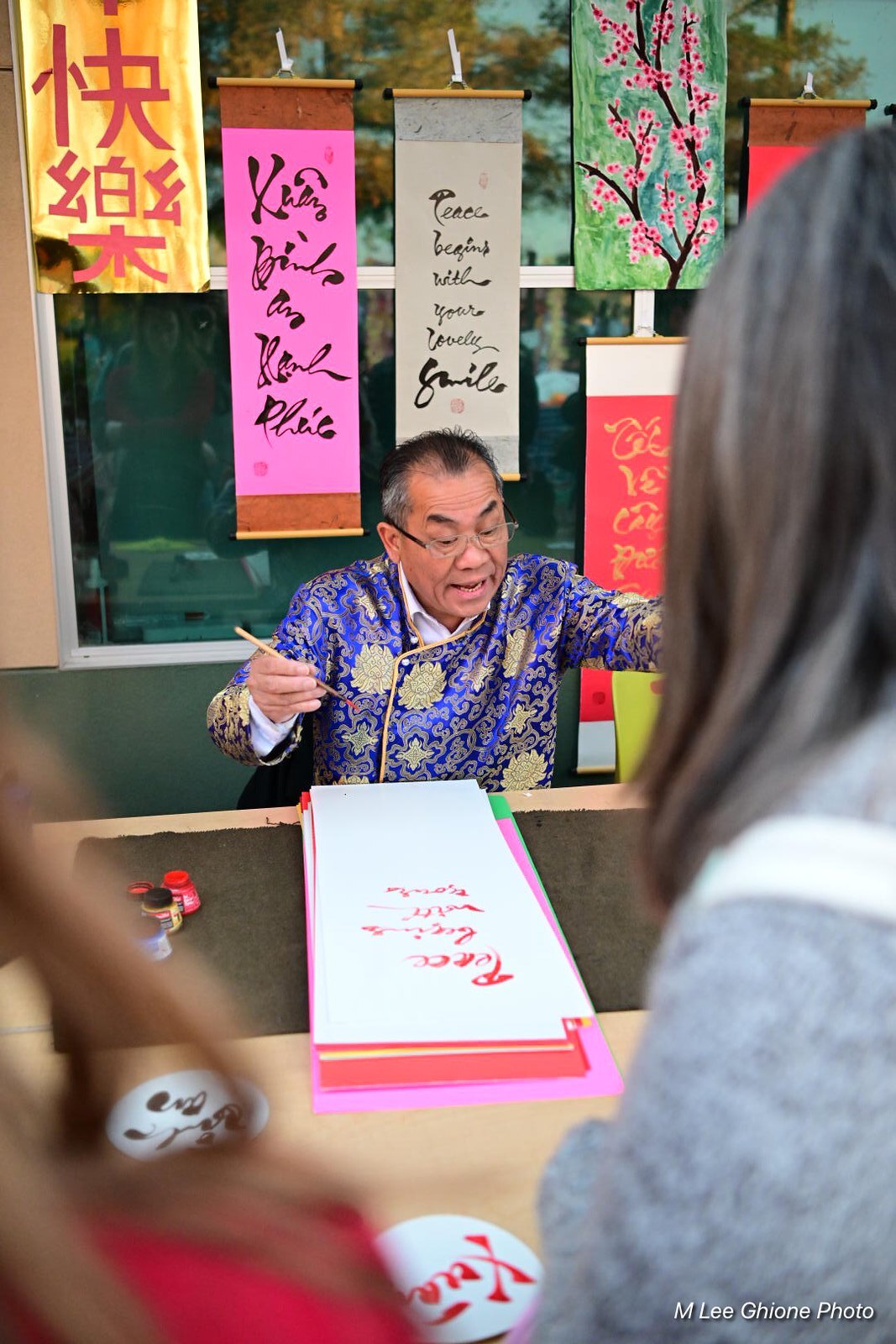The photograph showcases an older Asian man, possibly a calligrapher, seated at a table where he is deeply engrossed in writing on a long rectangular sheet of paper. He's adorned in an elegant, glossy blue shirt that buttons across the chest, accented with golden flowers. His short hair appears to be balding with black on top and gray on the sides, and he wears glasses. The man appears to be speaking while looking slightly to his right, away from the paper.

Directly in front of the camera, the blurry heads of two onlookers, one with long black hair and the other with long brown hair, can be seen, giving the perspective that the photo was taken from behind them. The room features a series of hanging scroll banners behind the man, including a vibrant array of colors such as yellow, pink, green, and red. One banner depicts cherry blossoms, while others are adorned with traditional calligraphy in various scripts and symbols, one of which includes classic Japanese characters in red text against a gold background.

The setting, indicated by these elements, suggests that the man may be performing or demonstrating calligraphy, possibly in a cultural or educational setting rather than a restaurant.